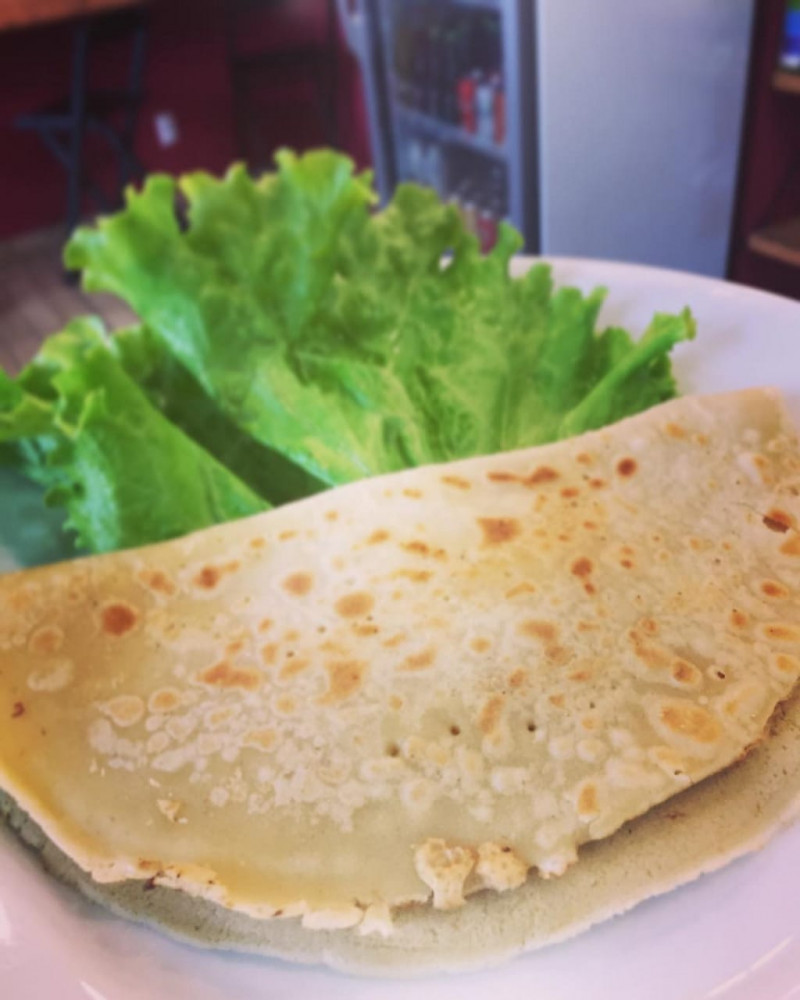The image features a detailed close-up of a white circular plate placed on a white table. The central focus is a crescent-shaped flatbread, possibly a taco or quesadilla, folded in half and showcasing brown marks indicative of being fried. Accompanying the flatbread is a slice of green lettuce, positioned next to it on the plate. The surface of the flatbread features small brown and white sparks. In the blurred background, a white refrigerator with a clear glass door is visible, housing various colored bottles—predominantly black, red, and white. The refrigerator suggests a kitchen or restaurant setting. The overall style is a realistic photograph with the objects in the forefront, sharply in focus against a softer background.